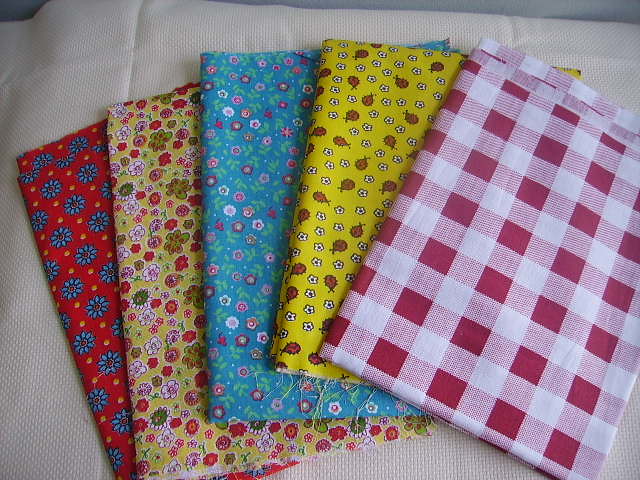This top-down photograph captures five freshly cut rectangular bolts of fabric, artfully arranged in a fanned pattern on a bright white sheet. Each fabric displays distinct color patterns and designs, with some edges showing slight fraying. From left to right, they are stacked in a manner that reveals a portion of each piece.

The fabric at the far left showcases a red background adorned with large blue flowers and yellow polka dots. To its right is a yellow cloth featuring a lively mix of white flowers, red ladybugs, and a subtle grid-like pattern interlaced with the floral design. The central piece stands out with a blue background, decorated with vibrant pink and purple flowers, complete with green leaves. Next is another yellow cloth, but this one is embellished with an abundance of pink, purple, or red flowers scattered across it. The final piece on the far right sports a classic red and white checkerboard pattern, reminiscent of a picnic tablecloth.

All five fabrics are laid upon each other, their layering and folded form revealing partial glimpses of each design, creating a visually appealing palette of colors and patterns in the brightly lit room.